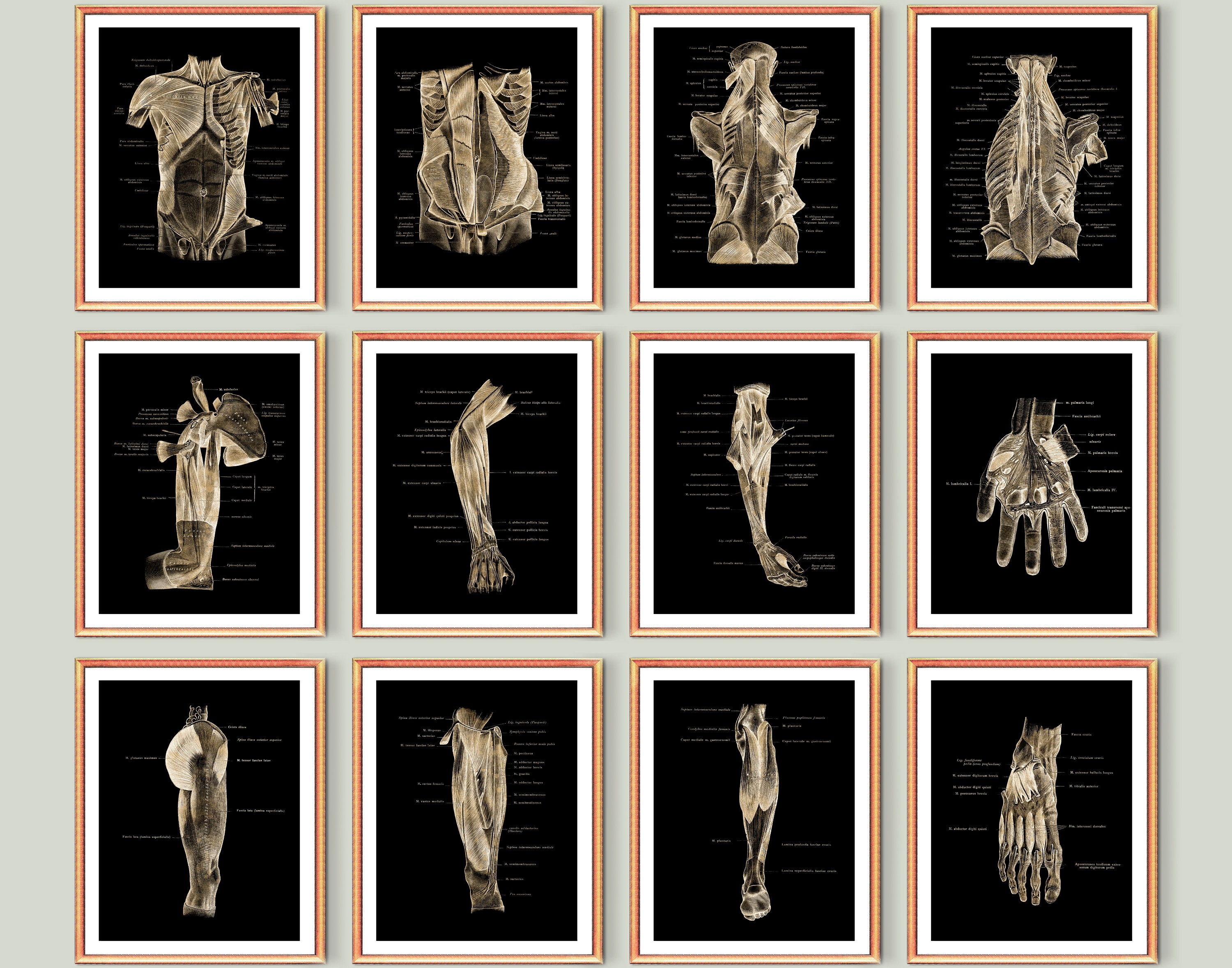The image displays a meticulously arranged collection of 12 anatomical illustrations, organized into three rows of four, each encased in a light-colored wooden frame with white matting. The illustrations stand out against a black background within the frames and are rendered in sepia tones. The arrangement forms a precise grid against a stark white wall, enhancing the neatness of the display.

Each illustration presents a detailed view of various human body parts, including the upper torso, ribcage, arms in different positions, hands, legs, feet, the back, and individual limbs such as shoulders, knees, and calves. Several illustrations exhibit surgical perspectives with the skin pulled back to reveal muscular structures, organs, and other anatomical details. The images, possibly used for medical or educational purposes, might be something seen in a human anatomy or biology setting. Despite the high level of detail and labeling within the illustrations, the specific text is unreadable due to the image size.